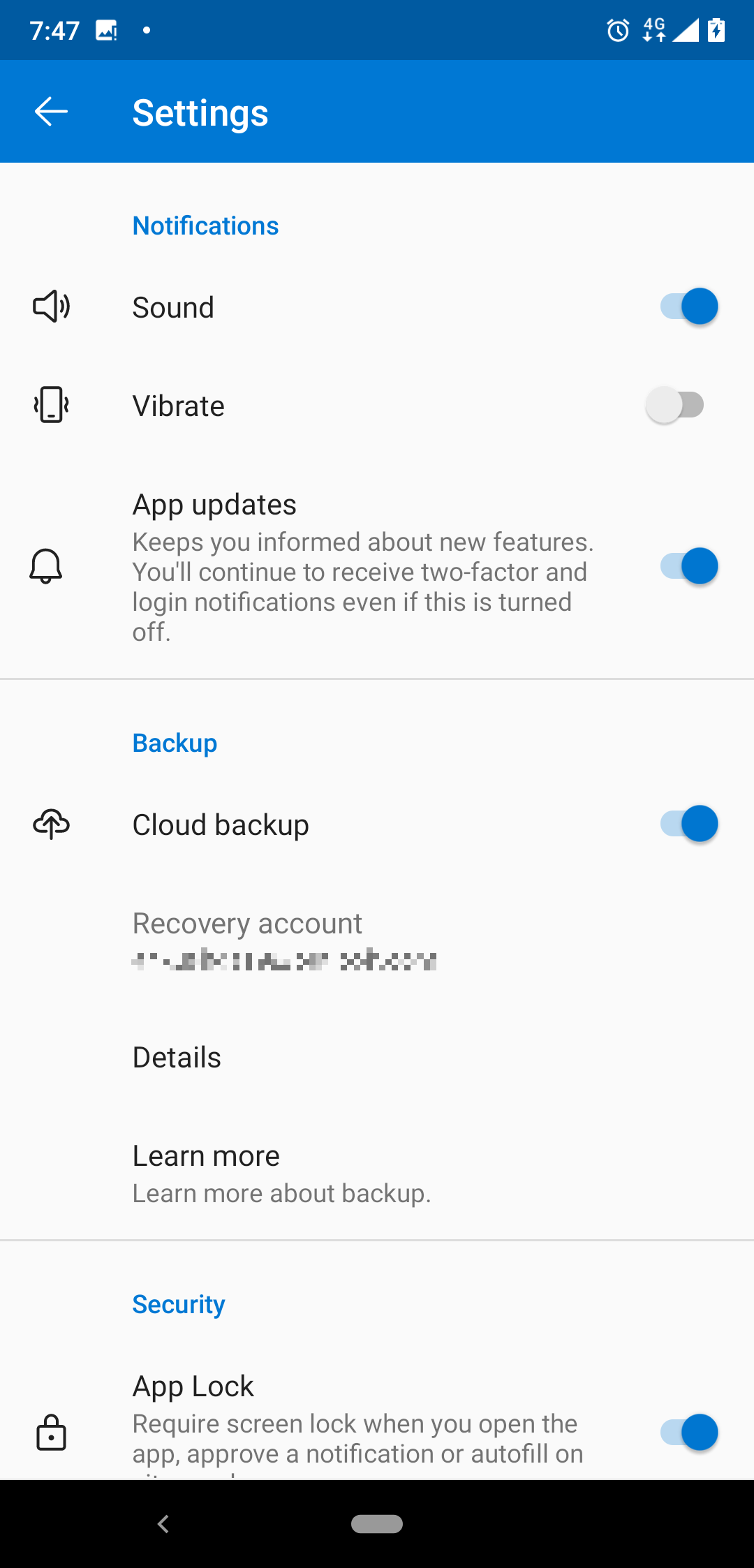This image is a screenshot from a smartphone. The background is predominantly white with a blue header at the top. In the header, the time is displayed as "7:47" in white font. To the right, there is a battery icon showing that the phone is charging, indicated by a small lightning bolt symbol in the center.

Beneath the top header, there is a slightly darker shade of blue header with "Settings" written in white font towards the left side. Next to it, on the far left, is a back arrow pointing to the left.

The main background of the settings page is white with various sections organized in blue and gray text. Below the medium blue header, the first section is titled "Notifications" in blue text, followed by gray text options: "Sound," "Vibrate," and "App updates."

The next section is labeled "Backup" in blue text, which includes options like "Cloud backup," written in blue, followed by "Recovery" and "Account," both written in gray. These are followed by "Details" and "Learn more."

The final section is titled "Security" in blue font and includes an "App lock" option.

To the right side of the image, each category has a toggle switch to turn the options on or off. The active options display a blue circle, while the inactive ones show a gray circle.